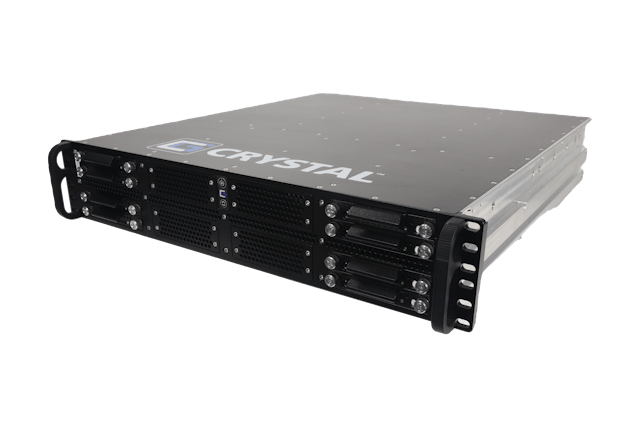The image depicts a professionally photographed server device branded as "Crystal" which is prominently displayed in white capitalized letters beside a blue rectangular logo with a white 'C'. The server is encased in a sleek black metal casing with a hard plastic front cover featuring vents and expansion slots secured by placeholder plastic plates with screws. The machine has small handles on each side of its face and side rails, facilitating its installation into a larger technical setup, such as a server rack. The polished, non-reflective black surface is punctuated with screws or rivets, adding to its sturdy, industrial aesthetic. The server stands out against a clean white background, emphasizing its sophisticated and professional design.